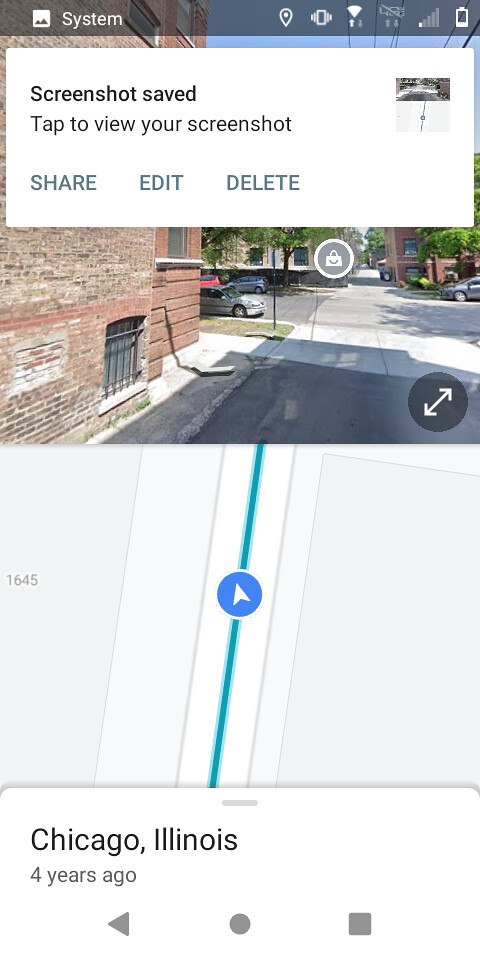The image is a detailed screenshot taken from a cell phone. At the top of the screenshot, the status bar shows multiple icons including a "System" label indicated by a small landscape square logo, a teardrop-shaped location tracker logo, a cell phone signal icon with lines emanating horizontally, vertical arrows representing data transfer, a Wi-Fi symbol, and a battery gauge icon. Below the status bar, a Google Maps screenshot is prominently displayed. Superimposed on the Google Maps image is a white notification rectangle, indicating "Screenshot saved" in black text with a small triangle icon. The notification prompts, "Tap to view your screenshot," and offers options for sharing, editing, or deleting the screenshot.